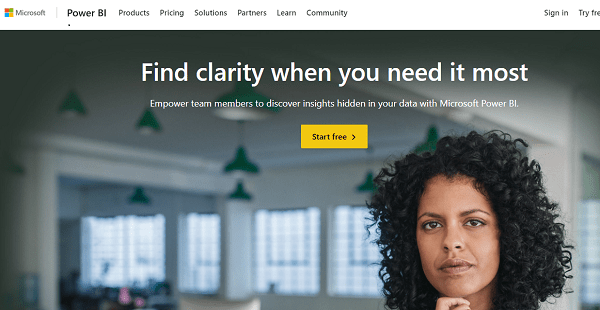The web page depicted is part of the Microsoft website, identifiable by the prominent Microsoft logo located at the top of a horizontal menu bar. The primary navigation tabs on this page include "Microsoft" (symbolized by the Microsoft logo, likely redirecting to the homepage), and sequentially from left to right: "Power BI," "Products," "Pricing," "Solutions," "Partners," "Learn," and "Community." On the far right of this menu bar are two call-to-action buttons: "Sign In" and "Try Free".

Currently, the "Power BI" tab is highlighted, indicating the content of the page is focused on this particular Microsoft technology. Below the menu, the main visual element features a woman with dark, curly hair and a serious expression. Above her, a headline reads: "Find clarity when you need it most. Empower team members to discover hidden insights in your data with Microsoft Power BI." Beneath this text, a prominent yellow button with an arrow invites users to "Start free."